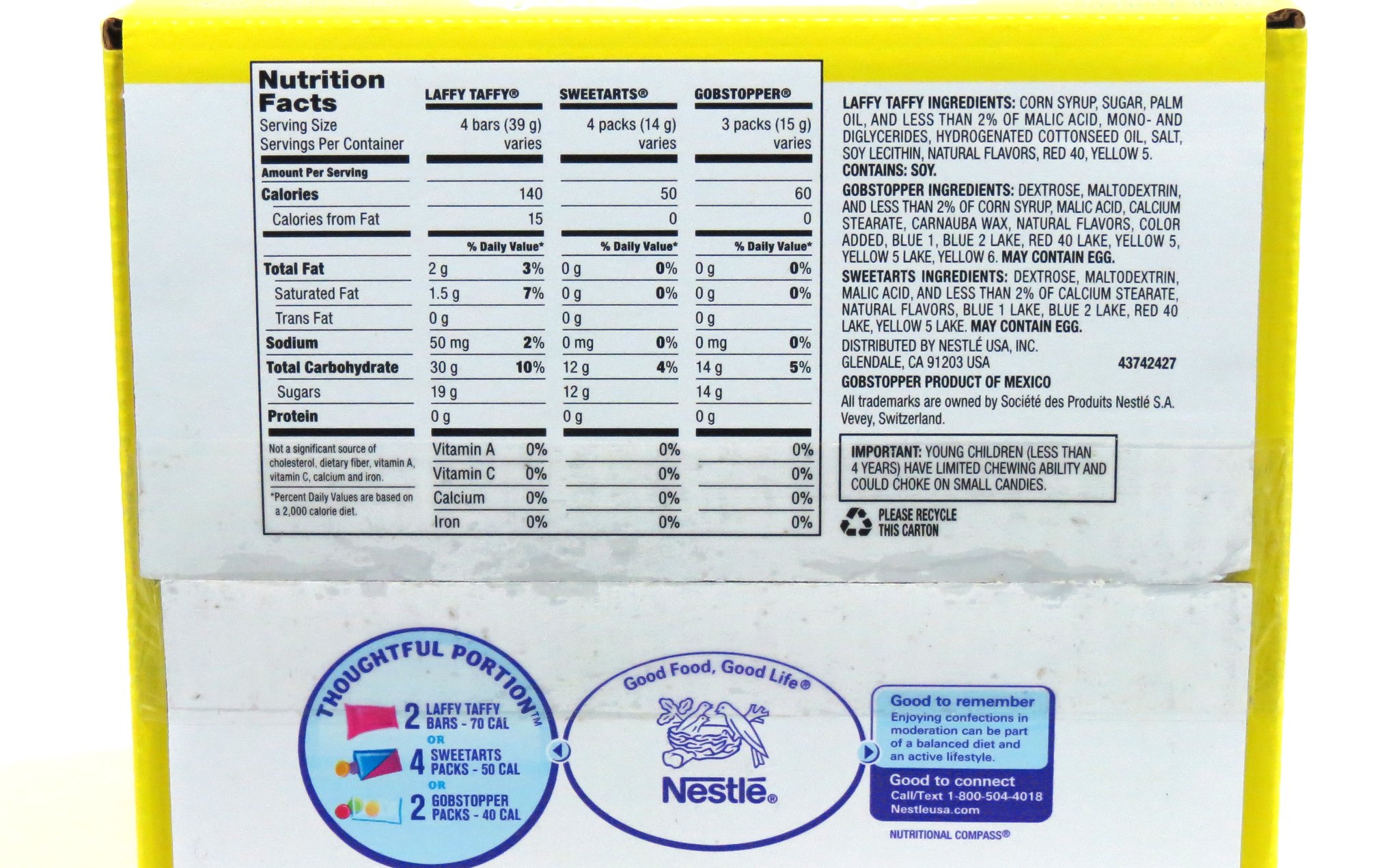A detailed photo of the back label of an assorted candy pack featuring Laffy Taffy, Sweet Tarts, and Gobstoppers. The label is predominantly yellow and prominently displays the Nutrition Facts. It lists serving sizes, servings per container, and calorie information for each type of candy: Laffy Taffy (4 bars), Sweet Tarts (4 packs), and Gobstoppers (3 packs). Below this, the ingredients for each candy are outlined individually: first Laffy Taffy, then Gobstoppers, and finally Sweet Tarts. The label specifies that the Gobstoppers are a product of Mexico. It also notes that all trademarks are owned by Société des Produits Nestlé S.A. Vevey, Switzerland.

An important safety warning is included, advising that young children under four years old may have limited chewing ability and could choke on small candies. There's also an environmental reminder to recycle the carton.

At the bottom of the label, three icons provide additional information. The left icon under "Thoughtful Portions" notes that two Laffy Taffy bars equate to 70 calories, four Sweet Tart packs to 50 calories, and two Gobstopper packs to 40 calories. The middle icon features the Nestlé logo with the tagline "Good Food, Good Life," illustrated with a bird in a nest. The right icon offers a reminder that enjoying confections in moderation can be part of a balanced diet and active lifestyle.

For consumer assistance and further information, there’s a contact section labeled "Good to Connect," providing a phone number (1-800-504-4018), a website (Nestleusa.com), and reference to the Nutritional Compass.